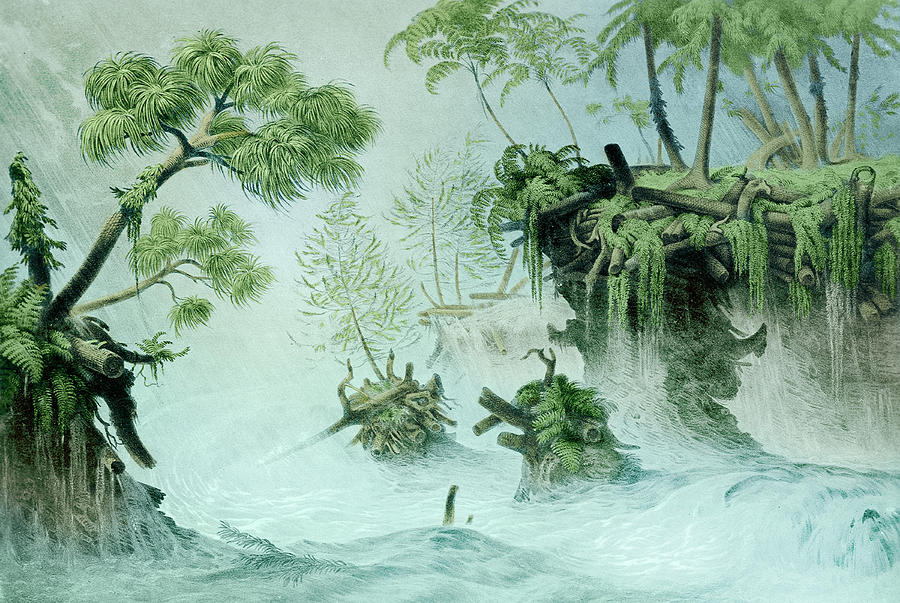This horizontal, extremely detailed color illustration depicts a dynamic prehistoric landscape in a fantasy style. At the heart of the scene is a turbulent, clear blue stream that originates from the center and flows towards the right, creating foam and light blue to white water as it churns. The left side of the image features an elevated, partially eroded landmass with a prominent tree leaning towards the middle, its roots gripping onto the remaining soil. On the upper right, another landmass is visible, populated by several palm trees and other types of trees, along with long strands of green moss draping into the water below. This area also shows signs of erosion, with broken logs and tree sections scattered, some of which appear to be part of what might have once been a dam, now destroyed and washed away. The background is filled with light tones of white, bluish-green, and hints at rough weather, with the wind adding to the sense of turmoil. The overall impression is one of natural forces in action, gradually reclaiming and changing the landscape.